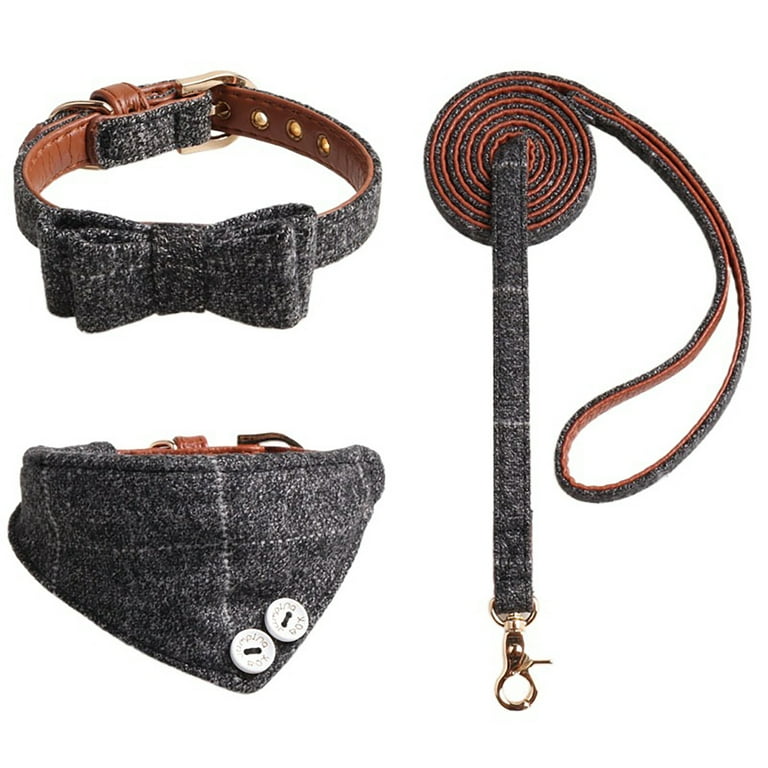This image features a set of three matching dog accessories displayed against a white background: two collars and one leash. All three items are crafted with a base of brown leather and are overlaid with a charcoal gray, checkered cloth. The upper left corner of the image shows a dog collar adorned with a bow tie, made of thicker cotton material. Below it is another collar with a bandana-shaped kerchief, featuring two white buttons at the far right tip. To the right of these collars is a rolled-up leash, with its handle protruding on the right and the clip section visible down the middle. The leash shares the same two-ply construction and checkered fabric design as the collars, making this a coordinated set.